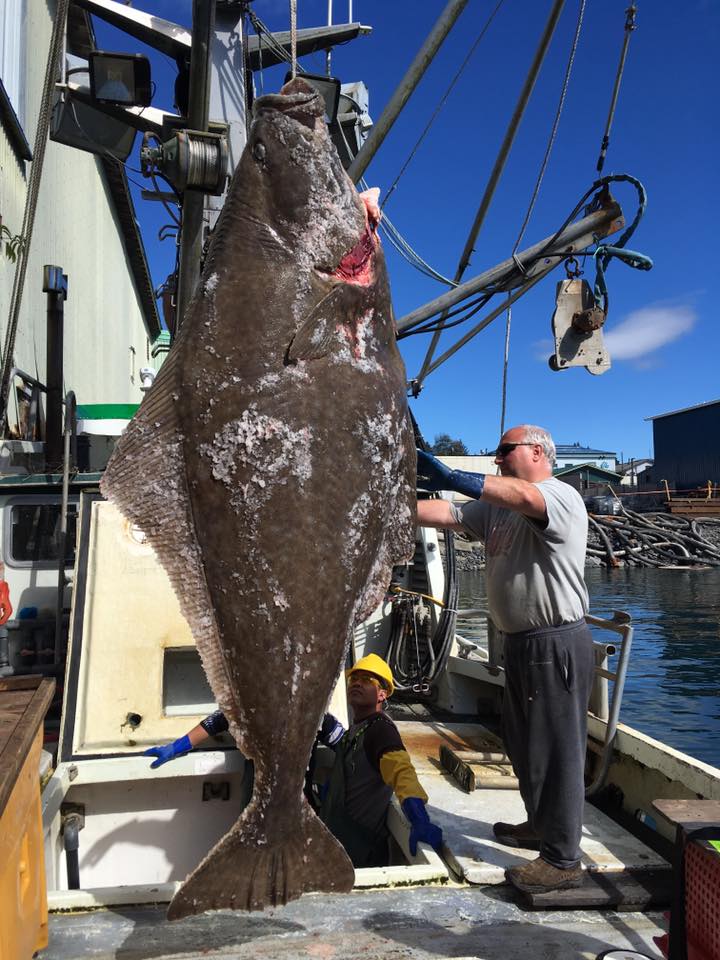This photograph, taken from the interior of a fishing ship, captures an expansive, dark brown fish hanging prominently by hooks in the center of the image. The fish, potentially a tuna, is enormous, appearing to be at least twice the size of the man touching it. This man, standing on the right side of the fish, is an older person with gray hair, dressed in a gray t-shirt tucked into black sweatpants, brown boots, and dark blue gloves. He is also wearing sunglasses and is facing the fish. Below him, the grayish-white deck of the boat is visible.

To the right of the fish, there are various wires, rods, and extensions scattered around the ship. Near the fish, emerging from the doorway on the deck, are two other men. One, partially visible, wears a yellow hard hat, glasses, a black and yellow jacket, and blue gloves. The second man is mostly obscured by the fish's tail, with only his arms visible as he steadies himself while climbing up.

In the background to the right, the blue water stretches out, reflecting sunlight on this bright, sunny day. Distant buildings line the shore, with the top of a single tree peeking above one of them. The sky above is a vivid blue, adorned with a few scattered white clouds, and the sunlight casts shadows that fall away from the viewer's perspective.